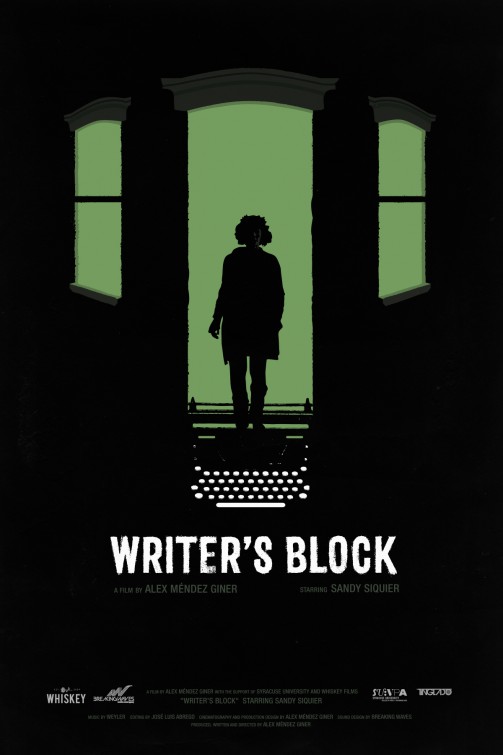The image appears to be a striking movie poster for a film titled "Writer's Block," directed by Alex Mendez Giner and featuring Sandy Sequier. Dominated by black, the poster features a silhouette of a woman with long hair standing in the arch of a green illuminated doorway. Surrounding her on either side are two small, green-lit windows set against the dark backdrop. The woman appears to be standing atop the silhouette of an old-fashioned typewriter, its white keys distinctly visible. The title "Writer's Block" and the director's name are prominently displayed in white letters. Additional text, including the word "whiskey" in the bottom corners, is also in white, with some gray text too small to discern, hinting at perhaps a production company or other credits. This artsy and minimalist design emphasizes mystery and creativity, aligning well with the independent film aesthetic.